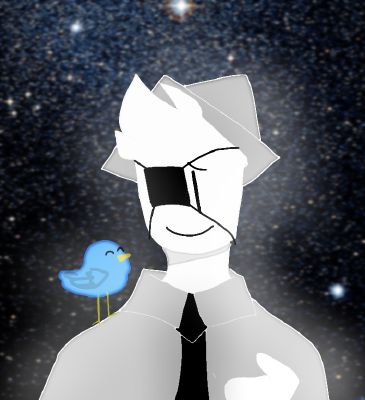This image is a detailed, abstract painting of a cartoon-like man set against a backdrop resembling the night sky. The man, depicted with stark white skin and white hair, wears a gray hat shaped like a triangle and an eye patch that obscures one of his eyes, creating a striking appearance. His mouth is a simple black line forming a smile. Dressed in a gray dress shirt and a black tie, the man appears static, yet engaging. Perched on his right shoulder is a blue bird with a yellow beak and long yellow legs, looking up at him intently. The background is filled with billions of star-like points of light, some larger and brighter than others, evoking the sense of looking through a powerful telescope into the vast, star-studded blackness of space. This painting, potentially created on a computer, merges simple, bright, and vivid elements to form a compelling, minimalist piece.